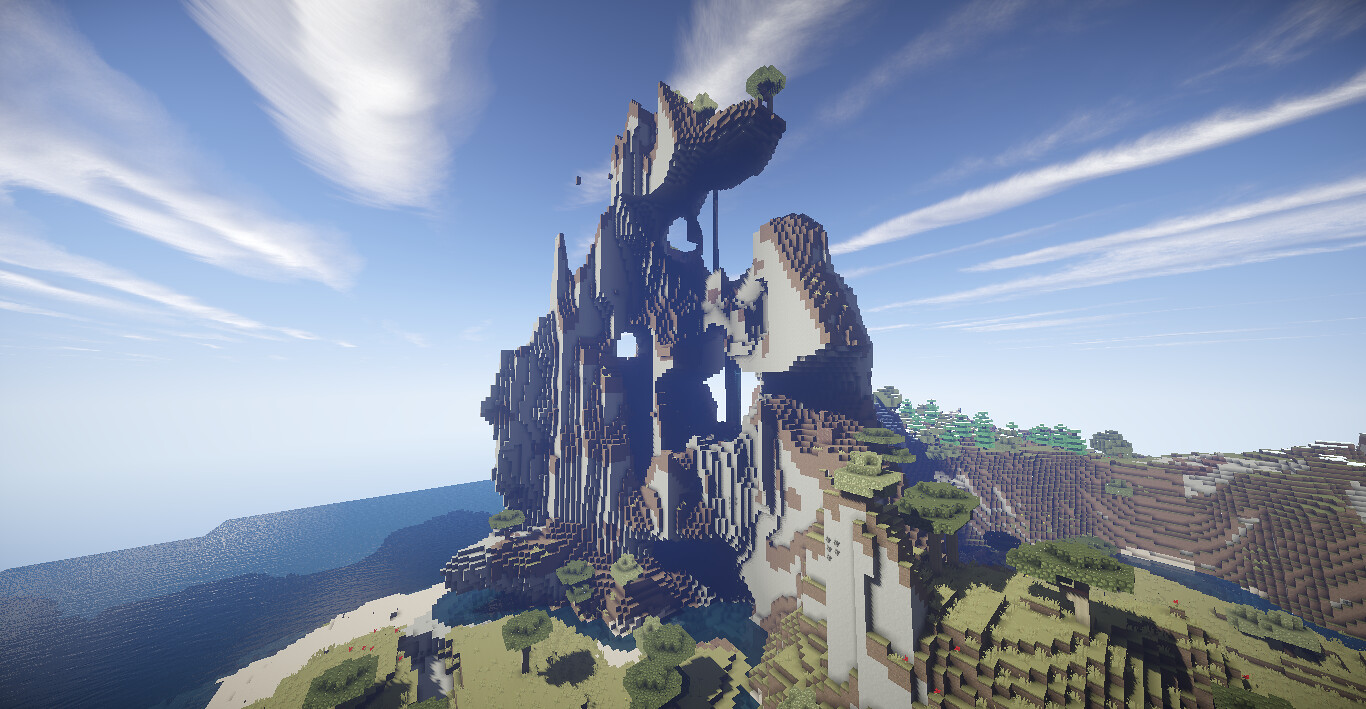This captivating image depicts a vibrant scene reminiscent of a Minecraft world, showcasing a spectrum of colors and intricate details. The bright blue sky, streaked with wisps of white clouds, stretches across the horizon. In the distance, an ocean of dual hues catches the eye, transitioning from a dark, deep blue to a lighter, more inviting shade. To the right, a lush grove of trees stands in contrast to the varied browns of the land that stretches below. Dominating the landscape is a towering, narrow structure that evokes the silhouette of a mountain or perhaps a monumental wall, reminiscent of the Great Wall of China, with its cream and brown tones. Above this structure looms a massive cliff, crowned with a solitary, majestic tree, completing the dynamic and detailed scene.